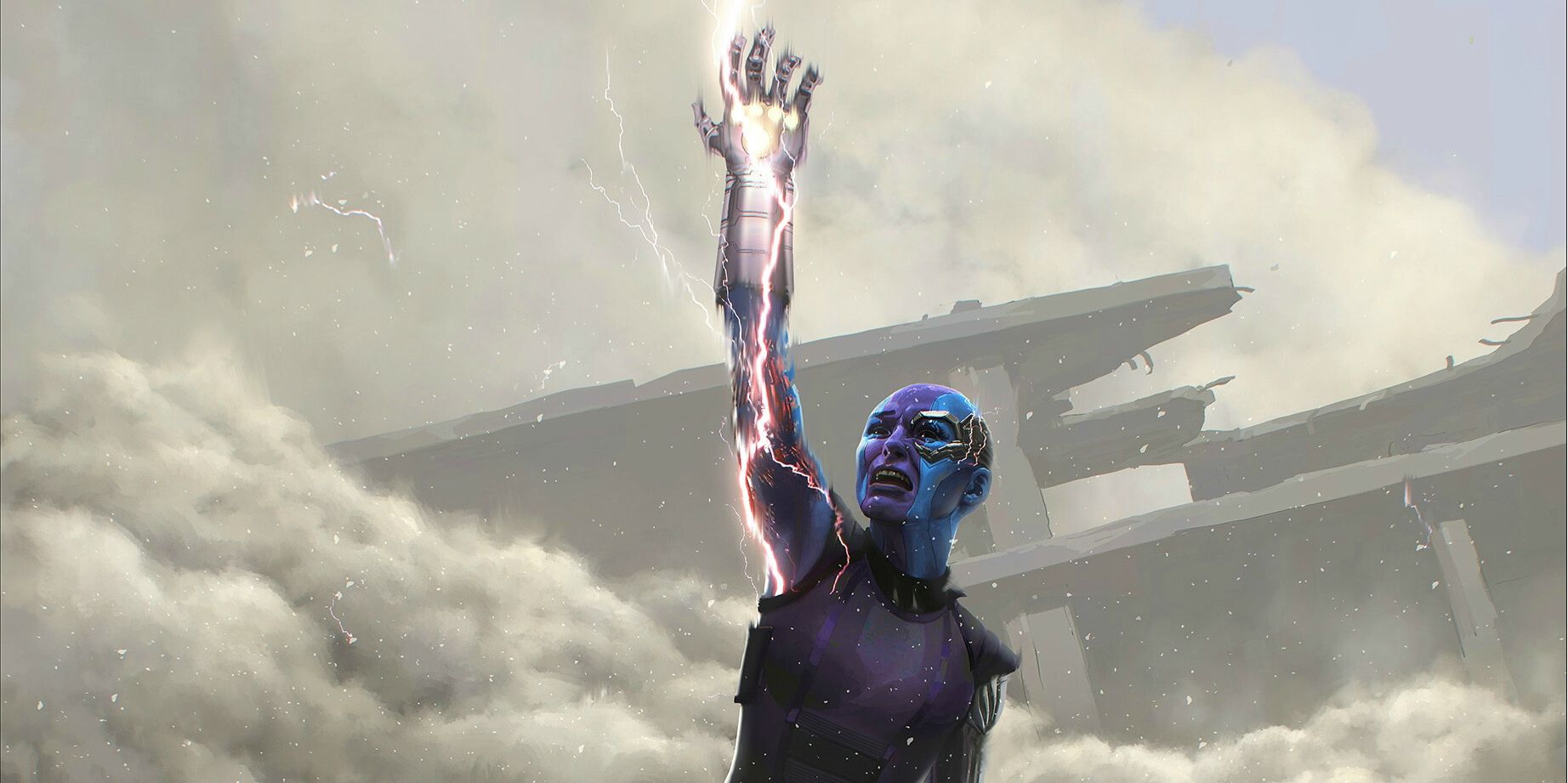The image is a detailed digital illustration or comic book frame showing a female android-like character, possibly from an Avengers film or video game. The central figure, a woman with a blue and purple face, wears a sleeveless black outfit with a purple tank top underneath. Her metallic right arm, clad in a silver glove, is raised towards the sky, channeling a white lightning bolt that travels through her arm, accentuating blue and red hues. She has a distressed expression on her face. In the background, a dark gray, partially collapsed structure, possibly a bridge or building, can be seen amidst swirling clouds or smoke. The sky is predominantly blue, indicating daytime, while the clouds or smoke hover near the bottom of the image, enriching the dramatic effect of the chaotic scenery.